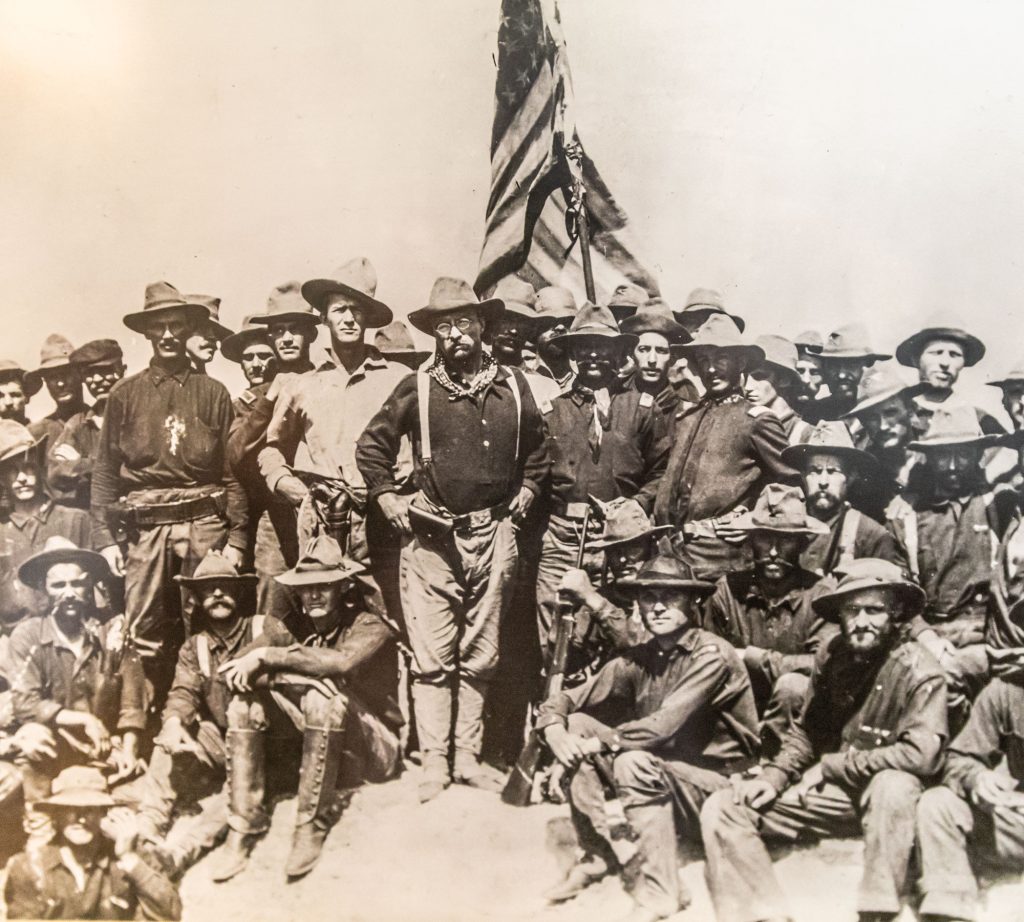This black-and-white sepia-toned photograph captures a historic scene featuring a group of men who appear to be Texas Rangers or Cowboys, possibly from the late 1800s to early 1900s, suggested by their attire and old model guns. Central to the image is a man with glasses, a large white handlebar mustache, a handkerchief tied around his neck, and wearing suspenders with a big belt buckle and gun holster. The men are adorned in straight-brimmed cowboy hats and leather jackets, indicative of their rugged frontier lifestyle. 

In the foreground, several men are kneeling, with one holding a rifle. Behind them, a large American flag is prominently displayed on a pole, adding a patriotic element to the composition. The group’s posed arrangement and their historical attire provide a striking glimpse into a bygone era of American history.